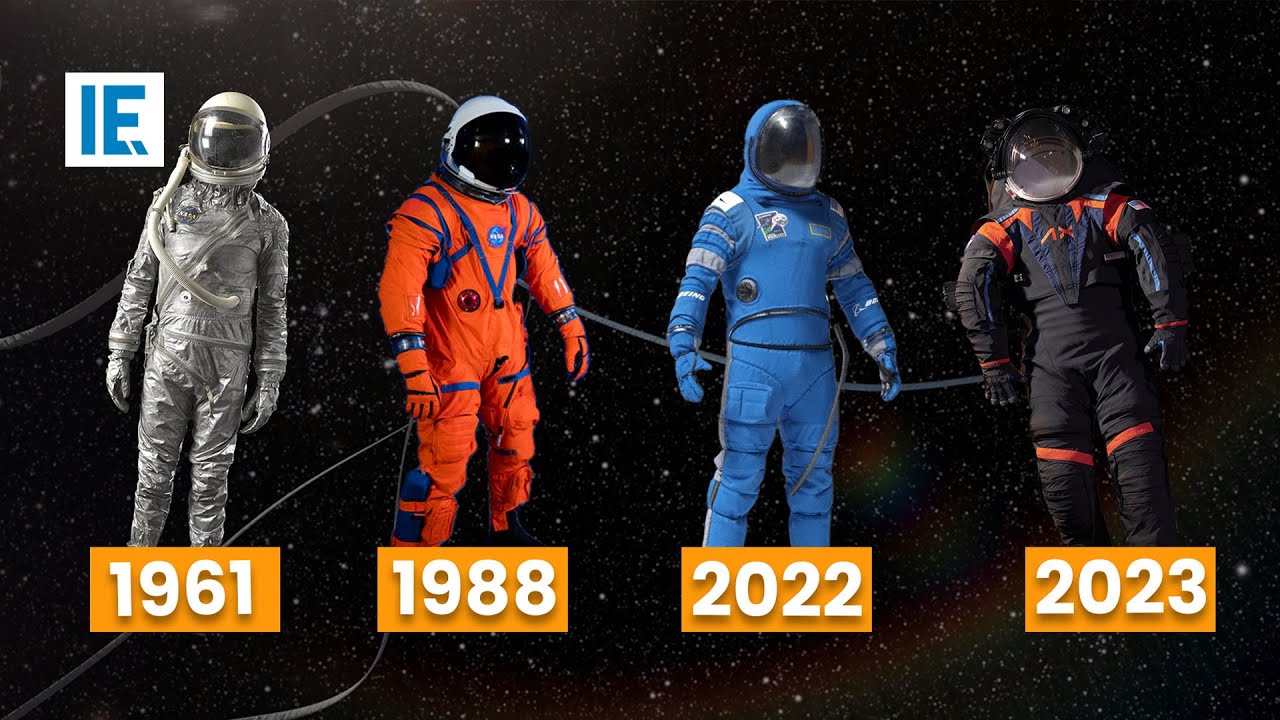The image is a rectangular illustration, wider than it is tall, depicting the evolution of spacesuits from 1961 to 2023 against a backdrop meant to represent space. The black background is dotted with small white stars, enhancing the space theme. 

In the upper left corner of the image, there's a white box with blue letters that say "IE."

The illustration features drawings or photos of four astronauts lined up from left to right, each wearing distinct spacesuits from different years. The first astronaut on the left is in a completely gray spacesuit with a gray helmet and gloves, labeled "1961." The suit includes several cables running behind it. This suit resembles those from the Mercury or Apollo eras.

To its right is a figure in a primarily orange spacesuit with blue details, a white and black helmet, and orange gloves, marked "1988." This suit has a design reminiscent of the Space Shuttle era.

Next is another astronaut in a blue and white spacesuit with a blue helmet and gloves, under which is the label "2022." This suit has a clear modern look.

The fourth figure on the far right is dressed in a black and orange jumpsuit with a black and white helmet and black gloves, labeled "2023." The cables running behind each astronaut tie all the suits together, signifying their connectivity.

This detailed illustration clearly contrasts the differences in spacesuit design and technology from 1961 to 2023.